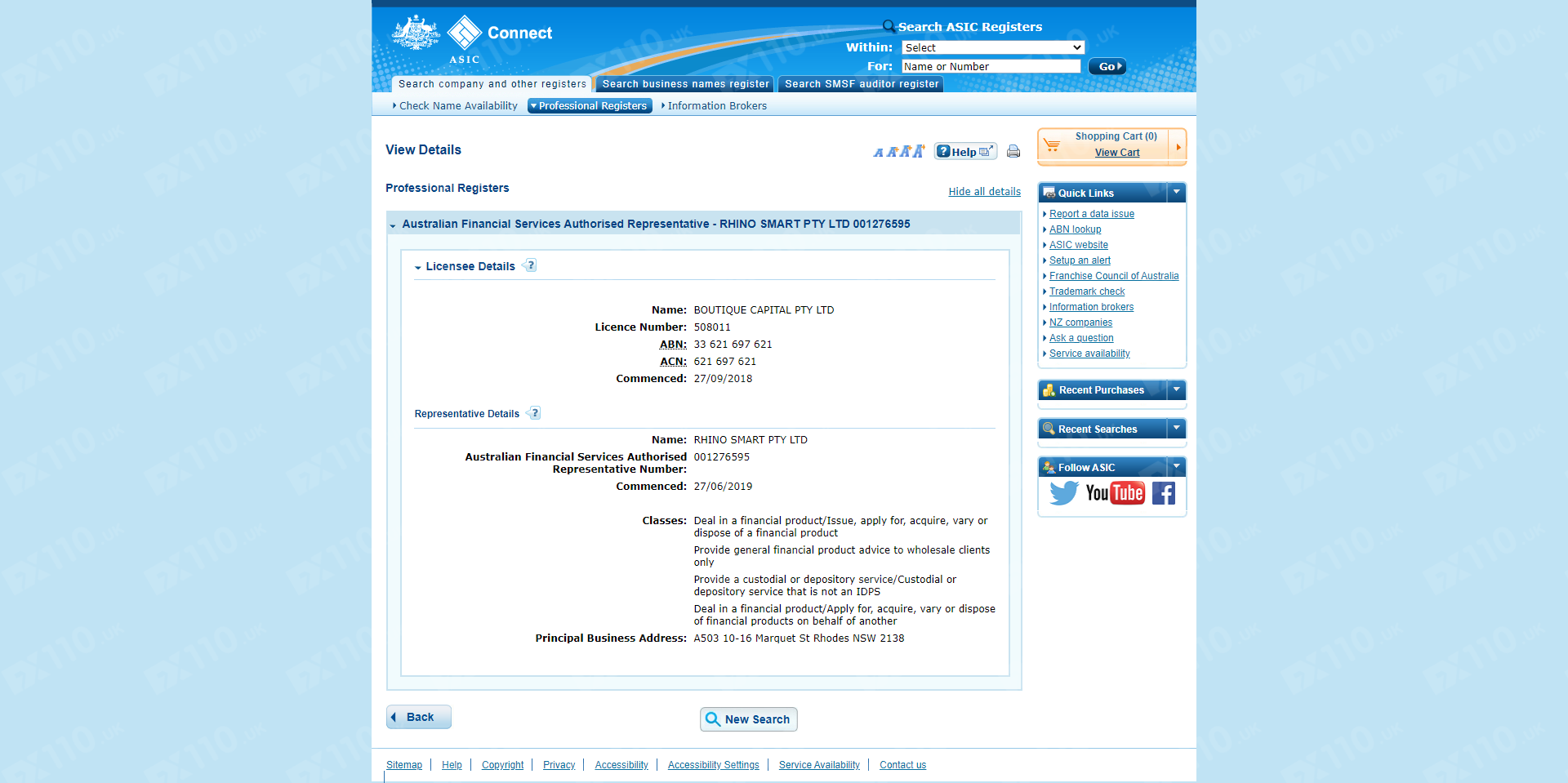A website interface for ASIC registration is displayed, featuring a vertically bracketed search engine positioned centrally against a light blue backdrop. At the top, a series of symbols are present, including bird icons and a lattice-like diamond shape, followed by the label "ASIC ASIC." To the right, the word "Connect" is prominently displayed, while the phrase "Search ASIC Registers" is presented in white text.

Below, a format dropdown box labeled "within" allows users to refine their search criteria by name or number, accompanied by a "Go" button. The interface includes three tabs: "Search Company and Other Registers," "Search Business Names," and "Search SMSF Auditor Register." Currently, the "Search Company and Other Registers" tab is active.

On the far left under the "Search Company" section, users can check name availability. Additionally, there's a "Retail View Details" option below, leading to the "Professional Register" section. Here, a dropdown box offers selections like "Australian Financial Services," accompanied by detailed license information. This includes licensee name "Boutique Capital," license number, ABN number, ACN, commencement date, and other representative details including the principal business.

At the bottom, a "Back" button appears on the left with a "New Search" button centrally located. On the right side, quick links to six or seven recent purchases and recent searches are available, as well as options to follow ASIC on various social media platforms.